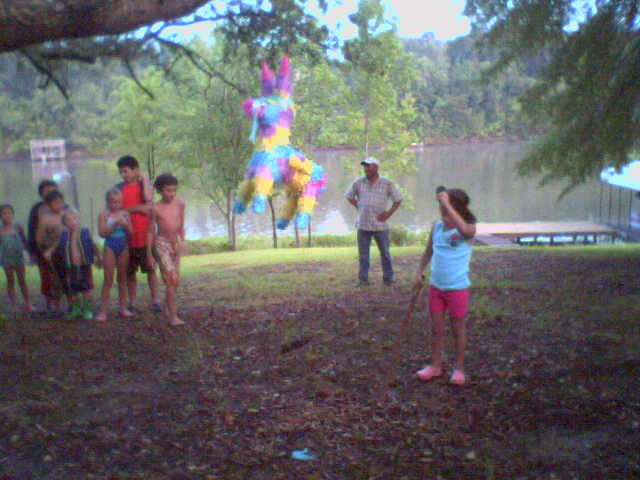In a sunlit, spacious backyard, a slightly blurry square photo captures a lively scene filled with children and a single adult. At the top, white and blue streaks mingle with a few tall trees adorned with lush green leaves, hinting it's a sunny day. The middle features a simple wooden fence enclosing the yard and a sizeable, multicolored pinata—blue, purple, yellow, and pink—suspending from a tree. This pinata, resembling a unicorn or donkey, is the focal point around which the action revolves.

In the foreground, a young girl stands on the right, poised with a bat, ready to take a swing at the pinata. She is clad in pink shorts, pink shoes, and a blue tank top, concentrating intensely on her task. A man in jeans, a white ball cap, and a short-sleeved button-down shirt stands slightly behind and to her left, supervising the activity.

To the left side of the frame, a group of children aged around 7 to 10 years, consisting of mostly boys and a couple of girls, forms a line, eagerly awaiting their turn. The ground below them is a mix of grass and scattered leaves, adding a touch of natural chaos to the otherwise well-organized setting. The fence and expansive backdrop suggest the backyard is quite large, with thickening tree foliage further in the distance enhancing the scene's depth.